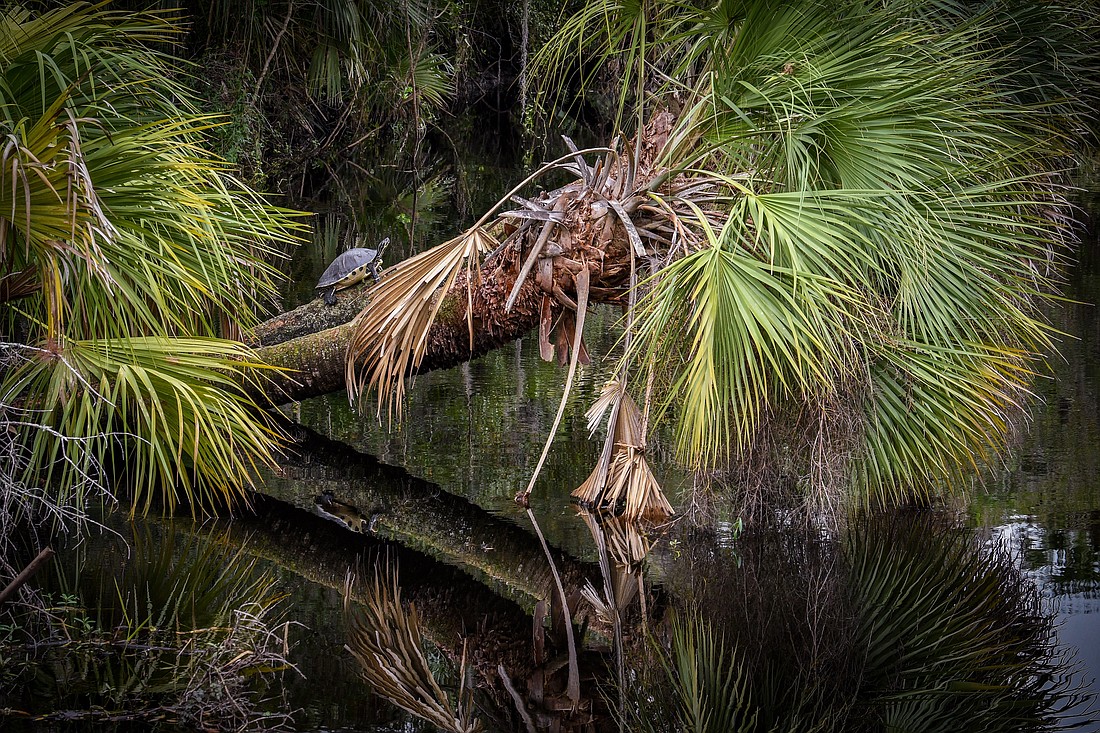In this captivating image, a fallen palm tree spans horizontally over a tranquil pond. A determined turtle is seen climbing along the sideways trunk, taking advantage of the tree’s new, more level position. Delicate, dead palm fronds dangle into the water, while the remaining leaves maintain their greenery, albeit with some brown edges. The turtle, almost reaching the top, suggests a slow, arduous journey along the trunk. The serene backdrop features other standing palm trees, whose reflections, along with the prominent mirror image of the fallen palm, create a peaceful, picturesque scene on the water's surface.